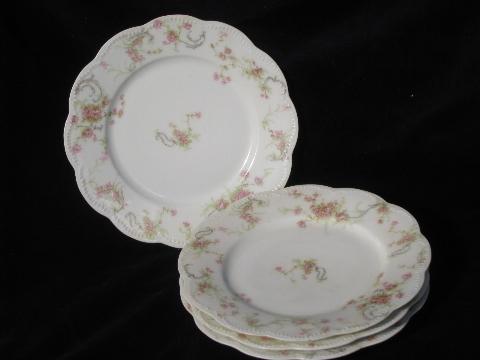The image captures a set of elegantly designed, vintage china plates set against a completely black background, enhancing their intricate details. There are four plates in total; three are stacked atop each other, while the fourth is positioned upright behind the stack, fully visible with its face turned toward the camera. The plates are white with a delicate, floral motif featuring pink roses and green vines placed centrally as well as along the perimeter. The edges of the plates are uniquely scalloped, with shallow ridges and small bumps, making them not perfectly round. This design ensures that food or gravy wouldn’t easily spill over. The lighting comes from the left side, subtly highlighting the contours and the floral patterns on the plates, which appear almost three-dimensional against the stark black background.